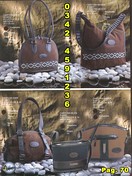The low-resolution, vertically oriented image appears to be a thumbnail photograph from a catalog or an online shopping website. It is split into two sections. The top section features two variations of brown handbags: one is akin to a woven crossbody bag and the other resembles a brown handbag, both adorned with decorative banding. The detailed craftsmanship makes them appear crocheted, although finer details are unclear due to image quality.

In the lower section, there are three additional handbags positioned on a bed of gray and white river rocks. These bags vary in color and design: one is tan, another brown, and the third appears to be either green or navy. Among them, a noticeable bag has a black top and chocolate brown bottom. An overlay of yellow text and numbers—0 3 4 2 4 5 9 1 2 3 6—runs horizontally across the image, slightly descending towards the middle-bottom section. Additional yellow text at the bottom right corner indicates "page 70."